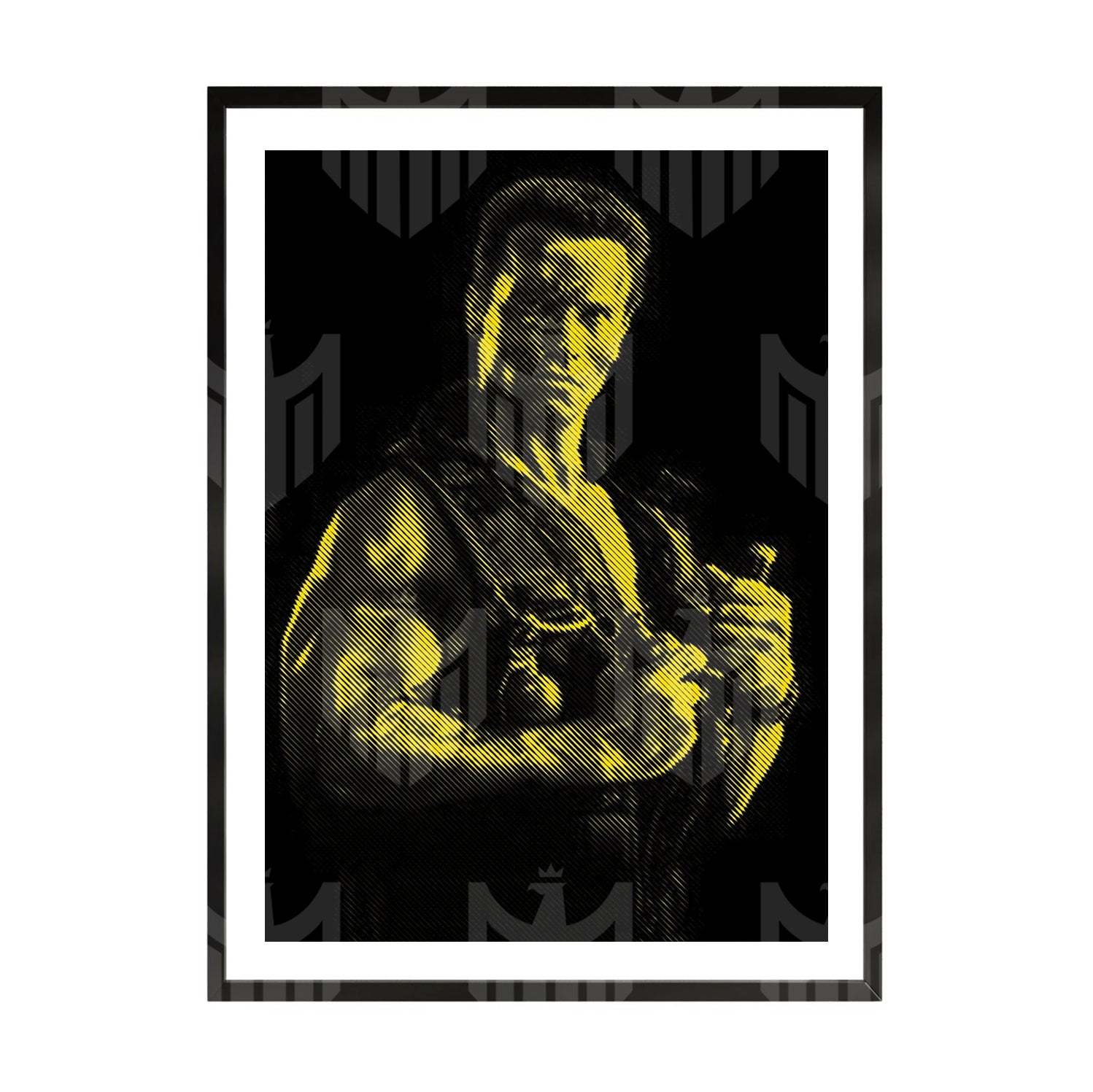The movie poster is a striking black-and-white vertical rectangular image featuring a young Arnold Schwarzenegger in a highly detailed and dramatic composition. Schwarzenegger, identifiable by his muscular physique and short, spiked hair, is depicted from the top of his head to his waist. He wears a sleeveless, army-like, puffy black vest, which exposes his well-defined biceps and is adorned with various tactical items, including a grenade strapped to his chest. In his left hand, he clutches a knife close to his chest, while his right hand holds another grenade, emphasizing his readiness for action. His body is slightly oriented to the right, though his piercing gaze is directed straight at the viewer, accentuated by darker paint smeared across parts of his face and body. The image is framed by an outer black border, followed by a white border, and backed by a gray and black background, enhancing the dramatic and intense atmosphere of the poster.